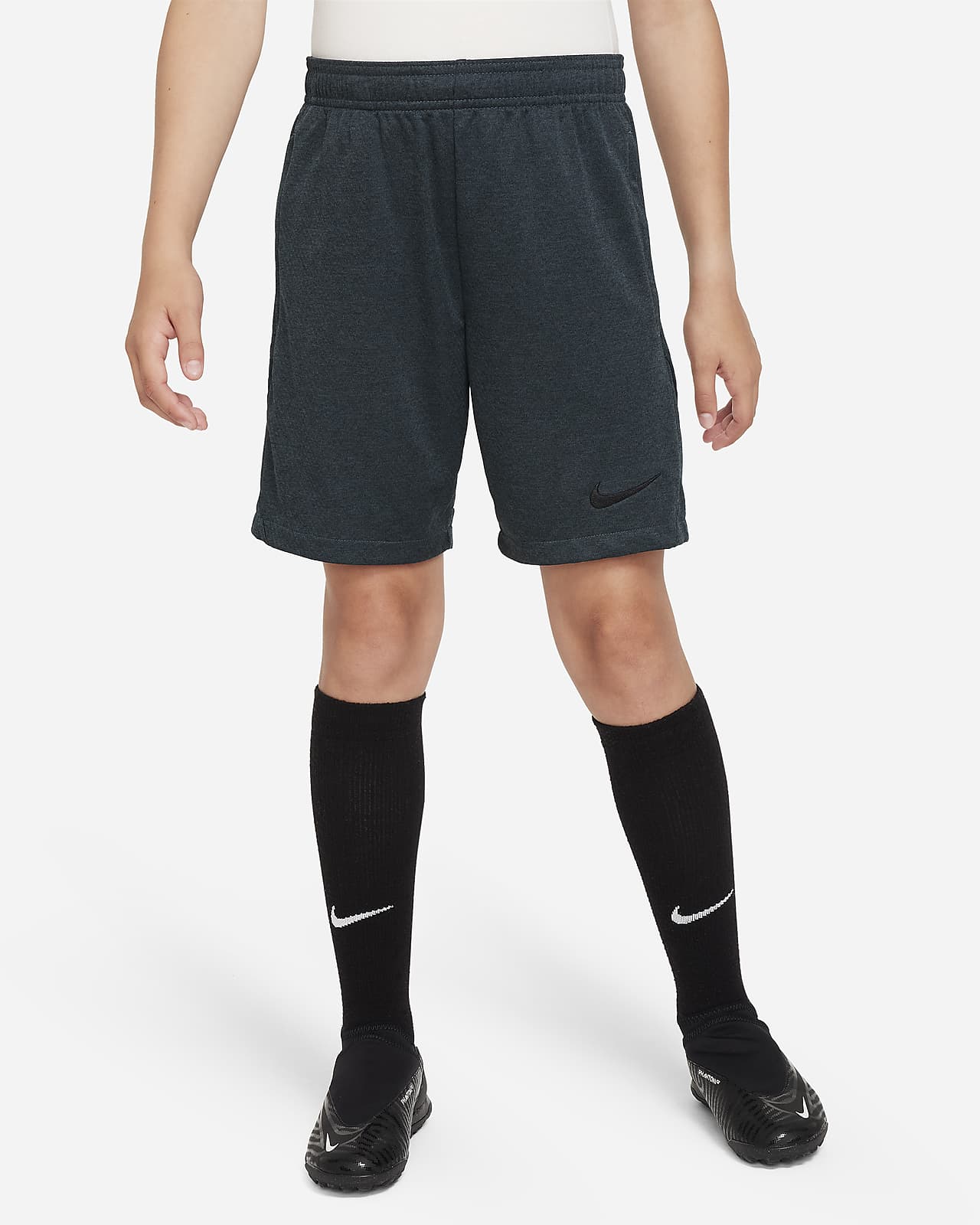In a minimalist studio with an all-white background and floor, a young male, approximately 14-15 years old, is modeling Nike apparel. The image captures him from the waist down, showcasing his athletic outfit. He is wearing a white shirt, partially visible at the top of the frame, tucked into dark navy blue Nike basketball shorts that reach just above the knee. Each item of clothing prominently displays the iconic Nike swoosh, with a black logo on the left leg of the shorts. His legs are adorned with long black Nike socks that extend to just below the knee, featuring a white swoosh on the shin. Completing the look, he sports sleek black athletic shoes with a shiny finish and a mixture of rubber and cloth materials. These shoes also bear the Nike logo on the outside and at the toe, emphasizing the brand's cohesive presence throughout the ensemble. The model's arms hang naturally at his sides, with the back of his thumbs facing the camera.